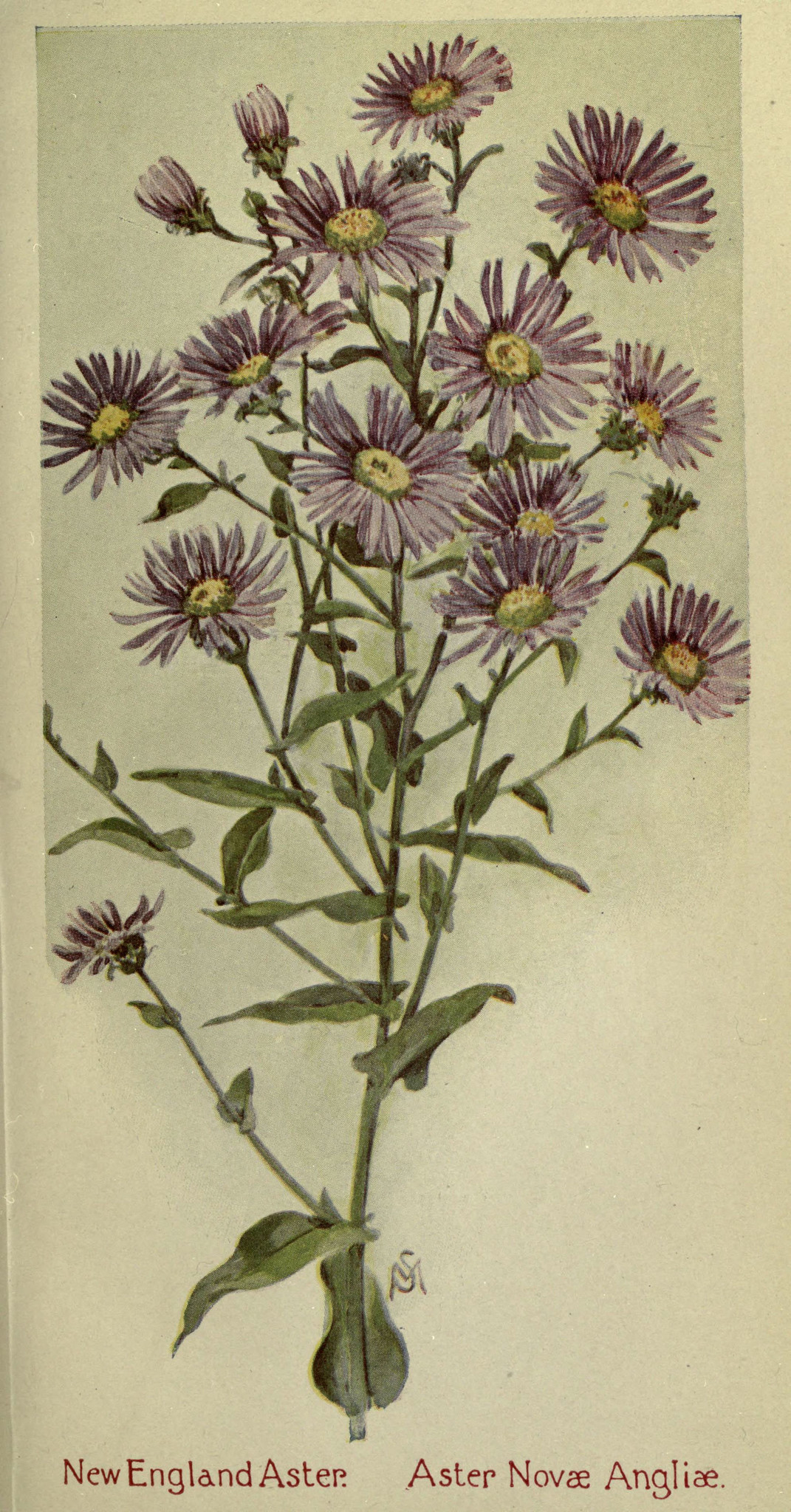This image depicts a beautifully detailed, vintage botanical print from the 1800s, showcasing the New England Aster (Astor Nova Anglaise). The aging of the paper is evident through its subtle yellowing, adding a touch of historical charm. The flowers, reminiscent of daisies, feature striking purple petals surrounding a greenish-yellow center. Each bloom is meticulously illustrated with careful attention to detail, capturing the delicate structure of the petals and stems. The print exudes an antique aesthetic, making it seem as though it belongs in an old nature book or displayed in a nature museum. The labels at the bottom provide both the English and French names of the flower, further emphasizing its classic botanical illustration style.